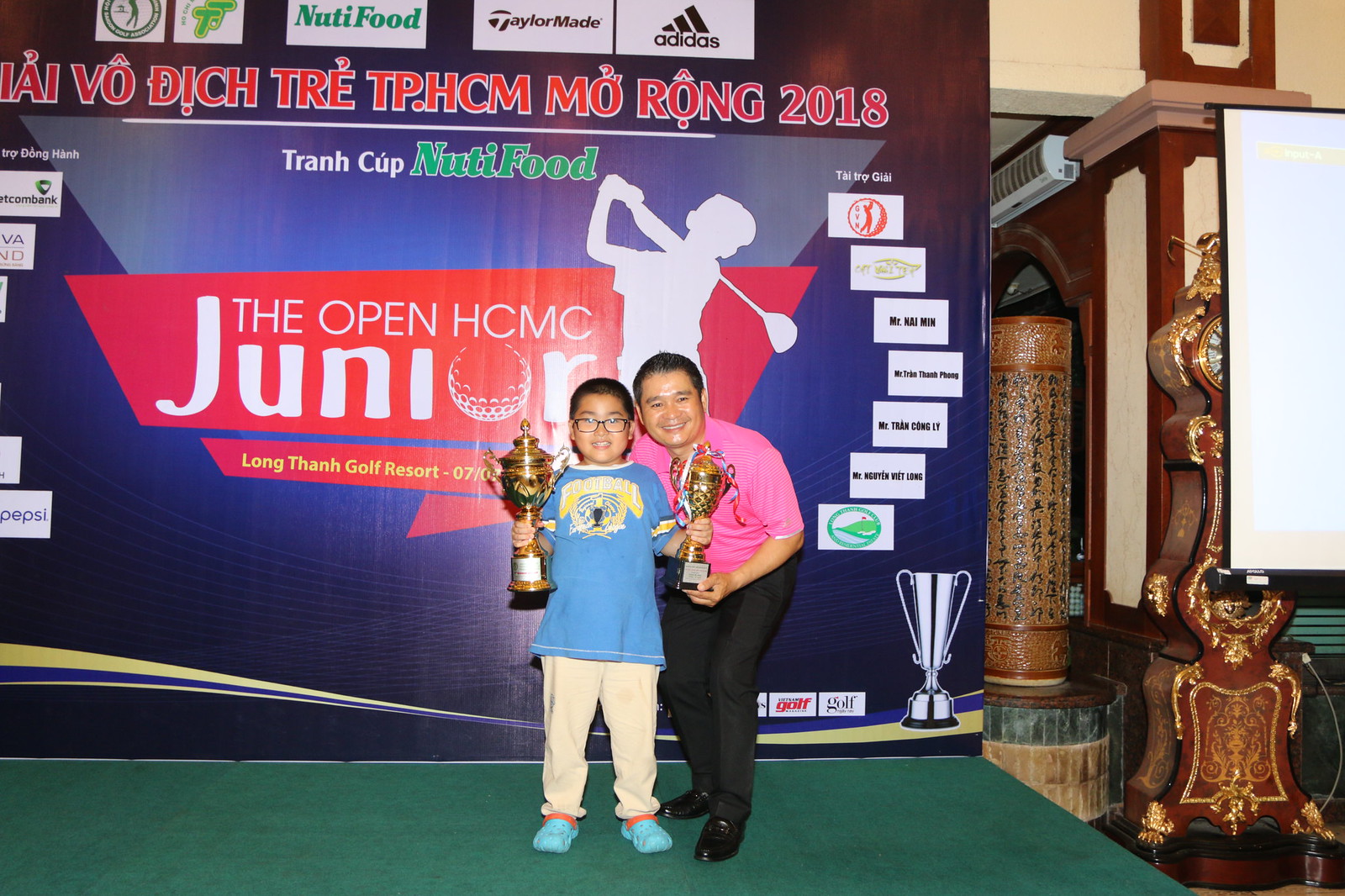In the photograph, a young boy and an adult man are posing indoors on a green stage, indicating a golf-related event, possibly the "Open HCMC Jr." tournament at the Longtone Golf Resort. The boy, wearing a blue shirt with yellow and white writing, white pants, and blue Crocs, is holding two large gold trophies — one in each hand. He is smiling and facing the camera, with glasses on. Next to him, the man, presumably older, is dressed in a pink shirt, black dress pants, and black shoes, and is also smiling into the camera.

The background features brown, tan, and white walls, adorned with items trimmed in gold, adding an antique feel possibly hinting at international origins. There is a wide banner in the background, predominantly blue and red, with multiple logos and text including "Tran Cup" and phrases like "The Open HCMC Jr." with a golf ball for the "O." Various sponsor logos such as Adidas, Pepsi, and Nudie Food are visible on the sign. A silver trophy is also seen at the bottom right of the image next to the kid. The event appears to celebrate a significant achievement in junior golf.